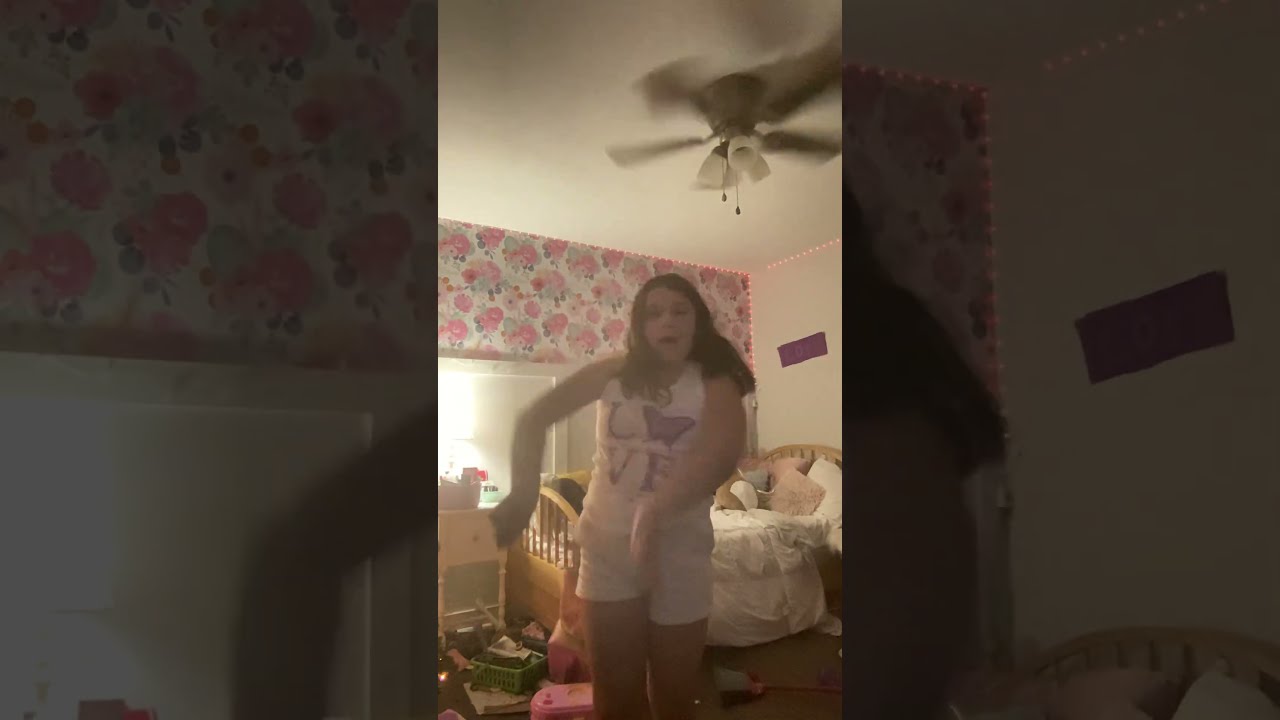The image captures a young girl dancing energetically in her cluttered bedroom. Her dark, long hair moves with her as she gestures with both arms in front of her, slightly blurred from the motion. She wears a white tank top with the word "LOVE" in purple, where a butterfly substitutes the "O," and white shorts. The room features a twin bed in the corner with a white comforter and pillows, alongside a nightstand with a lamp. Pink LED strip lights line the edge of the ceiling, casting a warm glow. A blurred ceiling fan with a clear light fixture spins above her. One wall is adorned with floral wallpaper in pink and green hues. The floor is scattered with toys and other items, contributing to the overall messy appearance of the room.